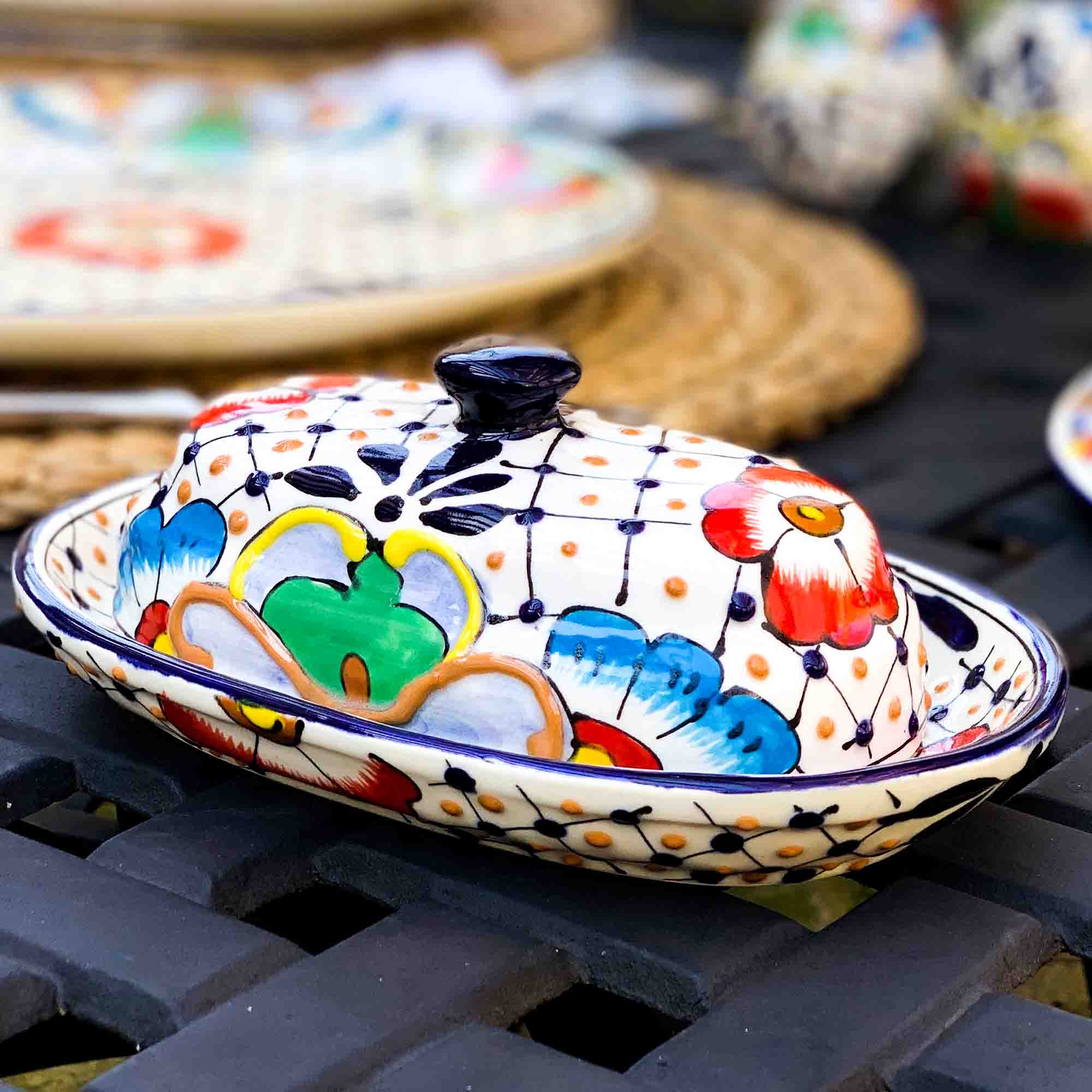This close-up photograph captures a handmade butter dish meticulously crafted from stoneware, resting on a heavy, blue-painted mesh table. The dish features a long, cylindrical bowl with a matching lid topped by a small black knob. The surface of both parts is adorned with an intricate woven pattern, enhanced by various vibrant colors and designs. Scattered across the dish are small reddish-orange dots and an assortment of painted flowers in hues of red, blue, green, orange, and yellow. The background is softly blurred, hinting at an array of matching handcrafted pottery, including plates and cups arranged on a wicker mat. The cohesive design extends to these pieces, indicating a cohesive and colorful set.